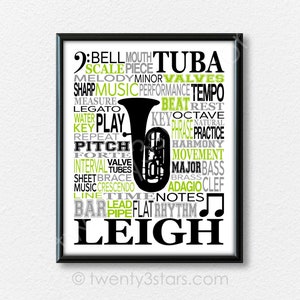This image features a framed piece of art with the watermark "23stars.com" at the bottom. The artwork has a light gray background and is centered around a small, animated black tuba or baritone instrument, depicted in silhouette. Surrounding the instrument are numerous musical terms written in varying font sizes and colors, including black, lime green, and gray. On the left side, words such as "bell," "scale," "melody," "sharp music," "measure," "legato," "water," "key," "play," "repeat," "pitch," "forte," "interval," "valve tubes," "sheet music," "brace," "crescendo," "line," "bar," "lead pipe," "time," and "flat" can be seen. On the right side, terms like "tuba," "minor valves," "performance," "tempo," "beat," "rest," "key," "octave," "praise," "practice," "harmony," "movement," "major brass," "bass clef," "adagio," "notes," "rhythm," and a black music note symbol are displayed. At the bottom of the image, the word "leigh" (spelled l-e-i-g-h) is prominently featured in bold black text. The artwork is encased in a thin black frame, likely made of plastic or wood.